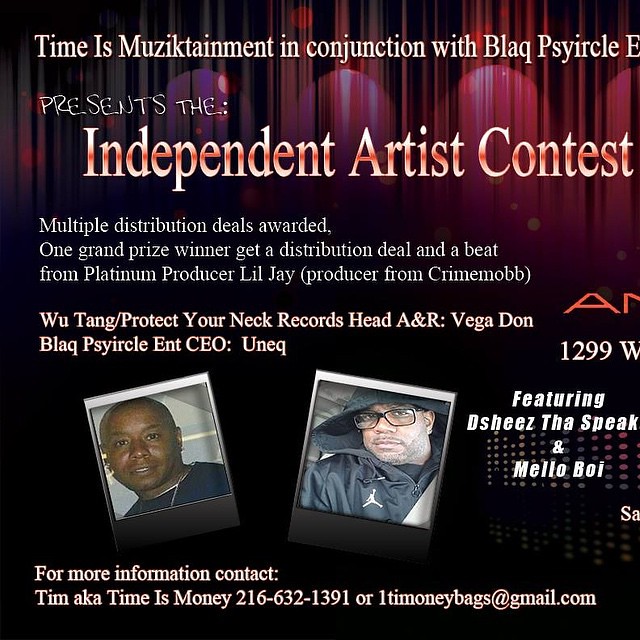This image appears to be an advertisement for an Independent Artist Contest organized by "Time Is Music Tainment" in conjunction with "Black Circle." The top of the flyer showcases a heading with the names of the organizing entities, followed by the announcement of the contest. The contest offers multiple distribution deals, with a grand prize featuring a distribution deal and a beat from platinum producer Lil Jay of Crime Mob fame. It mentions notable endorsements from Vega Dawn, the head A&R of Wu-Tang's Protect Your Neck Records, and Uneck, the CEO of Black Circle Entertainment.

The flyer includes two Polaroid-style photographs, presumably of key individuals involved in the contest, identified as Che the Speak and Mellow Boy. The background design features stage curtains illuminated by spotlights at the top, transitioning to a solid black towards the bottom. At the bottom of the flyer, it provides contact information for further inquiries, listing Tim, also known as "Time Is Money," along with a phone number and an email address, timemoneymusicbags@gmail.com. Even though the flyer has some spelling inconsistencies and partial cut-offs, these elements and figures prominently highlight its promotional intent.